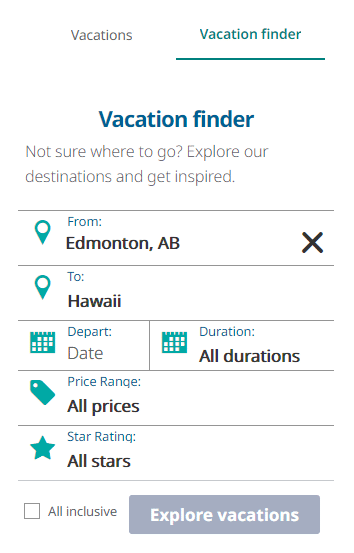The top of the website features the title "Vacation Finder" in a prominent blue font. Above this title, the left-hand side displays "Vacations" in gray letters, while the right-hand side shows a smaller, underlined "Vacation Finder." Directly below the central title, a phrase encourages users with the text: "Not sure where to go? Explore our destinations and get inspired."

A section starts with the text "From Edmonton, AB" followed by a black "X," and below it, a line reading "To Hawaii." A calendar icon accompanies the word "Depart," with a space provided for inputting the desired departure date. Adjacent to this section is another calendar icon labeled "Duration," with a drop-down menu featuring "All Durations."

Following this, there is a green price tag icon next to the heading "Price Range:" with fields where users can input their price preferences. Underneath this, "All Prices" is displayed in black text. 

A green star icon introduces the "Star Ratings:" section, which also allows users to select among "All Stars" in black text. Below this, a gray-outlined square with a white center offers an option labeled "All-Inclusive." 

Finally, there's a gray button with white text inviting users to "Explore Vacations."